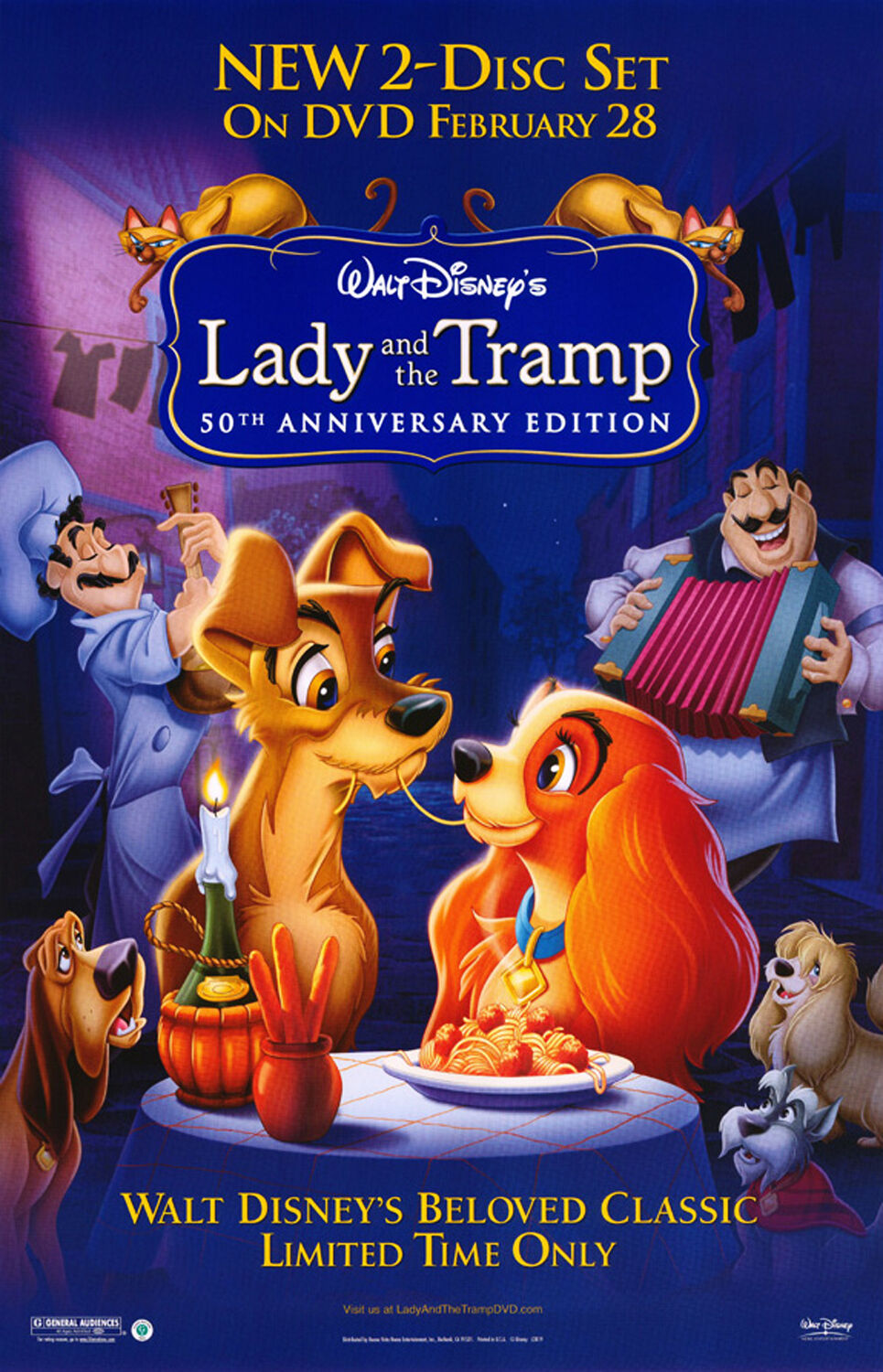This is an illustrated movie poster for Walt Disney's "Lady and the Tramp" 50th Anniversary Edition two-disc DVD set, predominantly featuring dark blue and yellow colors. At the top, in bright yellow lettering, it announces "New two-disc set on DVD February 28." Below this, two gold-colored cats sit above a dark blue placard with white text that reads, "Walt Disney's Lady and the Tramp 50th Anniversary Edition." The central image on the poster features the iconic scene of Lady and the Tramp sharing a strand of spaghetti, with a table set in front of them featuring a plate of spaghetti and meatballs, a glass wine bottle with a candle, and breadsticks. Surrounding the pair are three other dogs: one hound dog to the left and two others to the right, while in the background, a chef playing a guitar stands to the left, and a man playing a red accordion stands to the right. At the bottom of the poster, in yellow text, it reads "Walt Disney's beloved classic, limited time only," and there's additional yellow and white lettering below that, along with the Walt Disney signature in the bottom right corner.